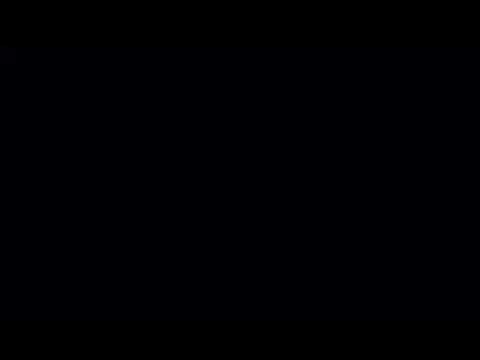The image displays a complete black rectangle or square, devoid of any other details, light sources, or textures. The black shape occupies the entire frame of the photograph and appears to be longer than it is tall, almost equilateral. It lacks any borders, shadows, or gradations, presenting a uniform dark surface. The screen itself is uniformly black, reminiscent of complete nothingness or a void, and retains a consistent coloration throughout without any hints of other colors or visible distinctions. The image is characterized by its simplicity and absolute darkness.